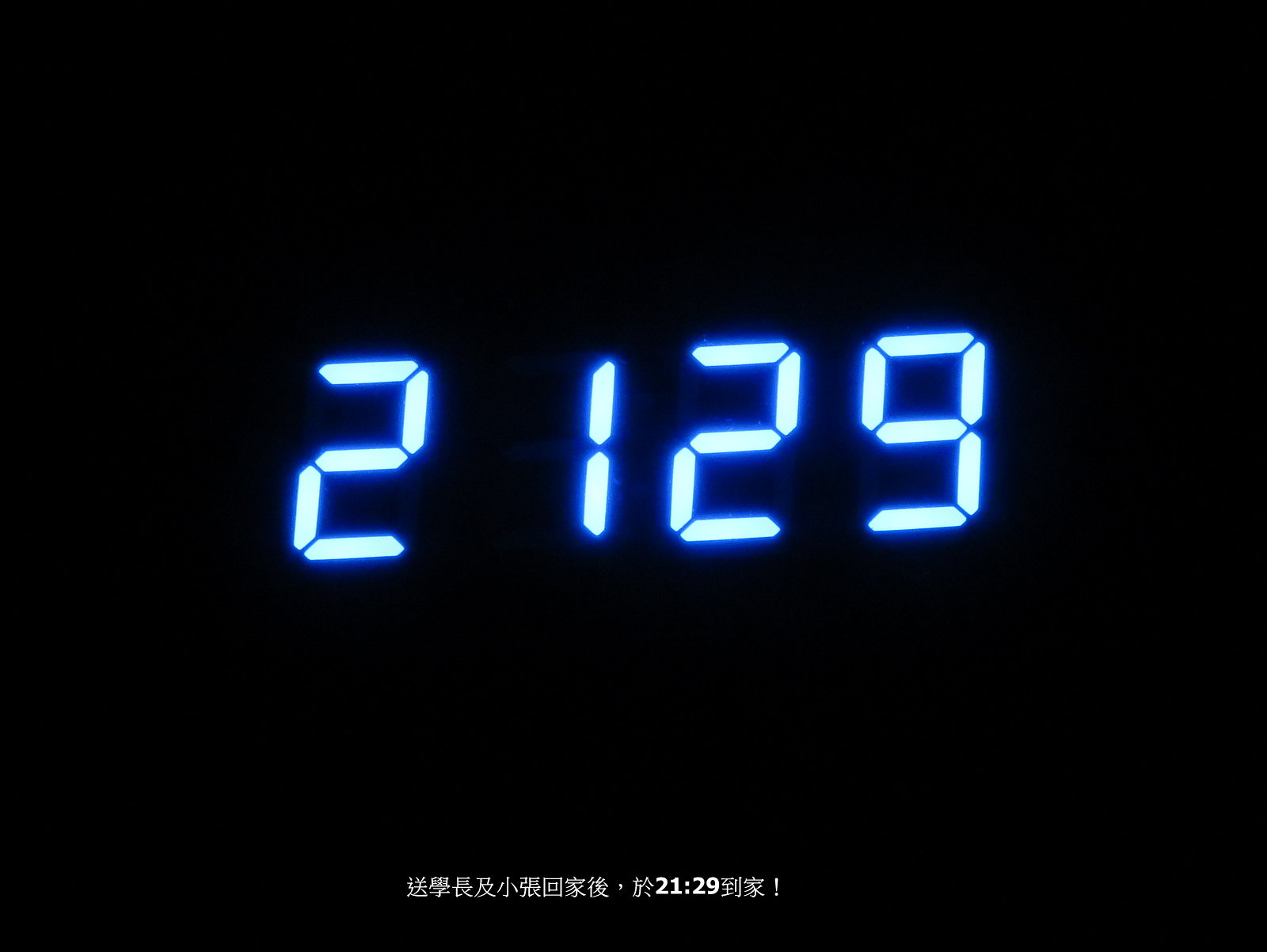The image is a close-up photograph of a digital clock set against an entirely black background, showcasing neon light blue numerals "21:29" in the center. The numbers are styled in the segmented manner typical of digital clocks, with noticeable separation between the digit "2" and the following "129." Below the time display, there is a strip of white text featuring non-English characters, likely Japanese or Chinese. Embedded within this script is the same time, "21:29," followed by additional characters and an exclamation mark. This arrangement suggests that the text provides some contextual information or message related to the time displayed.